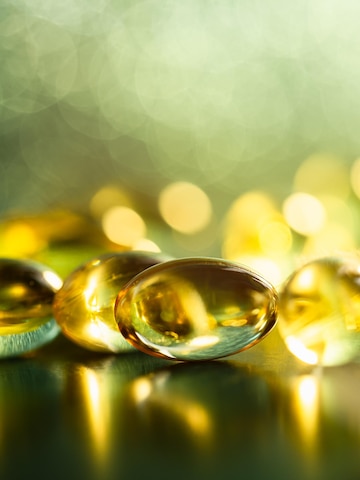This image is an ultra-close-up, artistic shot of what appear to be translucent, goldish-yellow gel capsules, likely vitamins or fish oil pills. The foreground features four prominently positioned capsules, each gleaming with reflections from a golden light source. They rest on a semi-reflective or metallic surface that mirrors their glow, adding to the scene's luminescence. The background is beautifully blurred using a bokeh effect, scattering the golden light into soft, circular orbs and introducing hints of green light. This bokeh technique creates an enchanting, almost ethereal backdrop that contrasts with the sharp clarity of the capsules. The overall color palette features dominant hues of gold, with green reflections adding depth to the image.